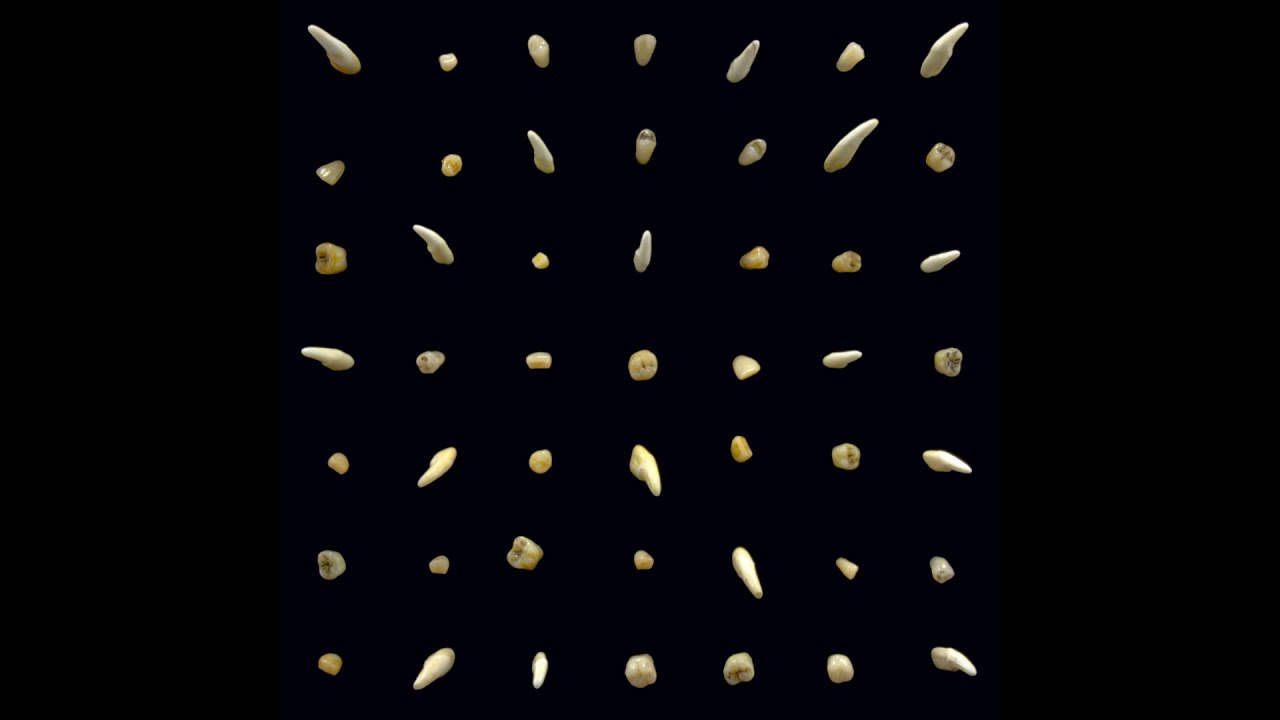The image displays a meticulously arranged grid of 49 shells evenly spaced on a flat black background, forming a perfect seven-by-seven square. Each shell, illuminated to reveal subtle variations, maintains a consistent distance from its neighbors, accentuating the grid's symmetry. The shells, varying slightly in shape—from elongated to spherical—predominantly exhibit a beige-ish yellow hue. Despite their uniform arrangement, these shells present an array of forms and tints that add a layer of complexity to the composition. The overall effect is a carefully curated collection, seemingly viewed from above, that contrasts strikingly against the dark backdrop.